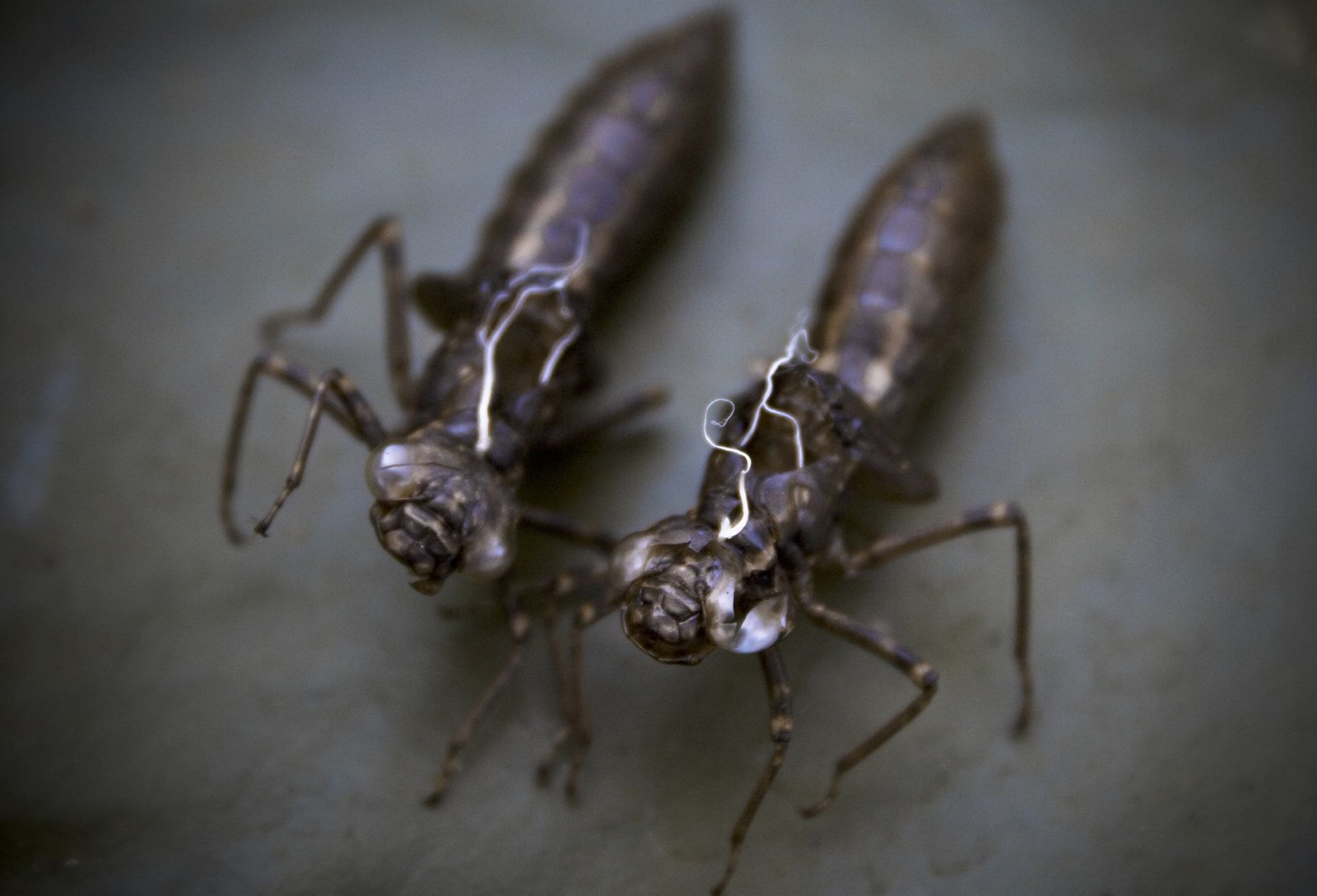This close-up image captures two brown insects with large, prominent eyes and six slender legs each. The insects are oriented towards the camera, appearing to lean on each other in a way reminiscent of a loose embrace, with one seemingly wrapping an arm around the other. Their bodies taper towards the rear, each ending in a pod-like structure that resembles a stinger, hinting at a possibly defensive feature. The insects are perched on a textured, brown-gray surface that offers a neutral backdrop, contrasting with their intricate, slightly unsettling forms.